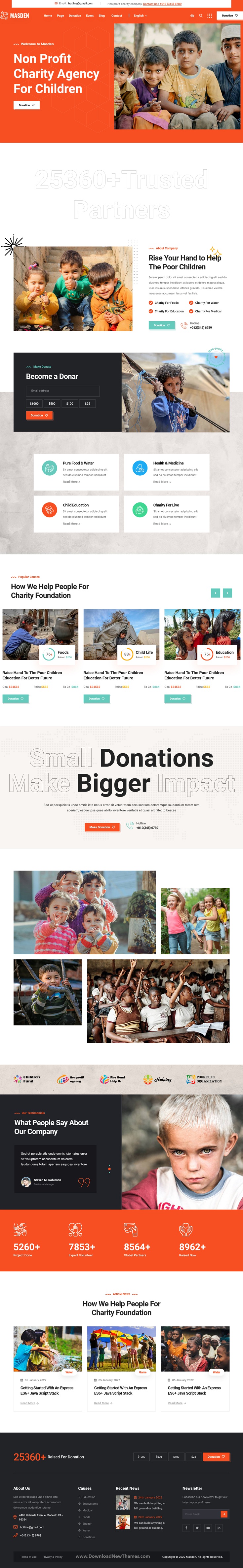The image features a complex layout with a variety of elements and color schemes organized across different sections. 

At the top is an orange rectangle, which contains a smaller white rectangle with unreadable text. Below the orange rectangle, another white rectangle is present with more illegible text. Prominently displayed is a phrase indicating a non-profit charity agency for children.

Underneath, there is a white section featuring an image of four children followed by another white area and a second image of three children. To the right of these images, there is some textual content accompanied by orange dots and a bluish-green rectangle. A black rectangle containing blue and white text is also present, followed by another orange rectangle with text.

Further down, on the right, an image of a child holding an unidentifiable object is seen above a gray rectangle. This gray rectangle includes four smaller white rectangles, each showcasing a different colored oval (bluish-green, orange, blue, and green) with text beside the ovals. In this section, there is both orange and black text, followed by blue text on the right-hand side. Three images, each with a white rectangle and illegible symbols, are aligned beneath these elements.

Three bluish-green rectangles are positioned near a light gray rectangle bearing the word "donations" in black, accompanied by more unreadable text. An area marked with the word "bigger" in black is followed by additional black writing, an orange rectangle with text, and more child images.

Toward the lower section, a gray rectangle contains symbols and black text, succeeded by a black rectangle with writings in orange and white, a white paragraph, and a symbol. Adjacent to this, another child image appears next to an orange rectangle with white text and symbols, and additional black text beneath.

Lastly, three more child images are present at the bottom with black text below them, followed by a black rectangle showcasing orange and white text. On the upper right-hand side, another orange rectangle is visible, paralleled by images positioned towards the center with accompanying text and some lighter gray bars. One of these bars contains an orange rectangle.